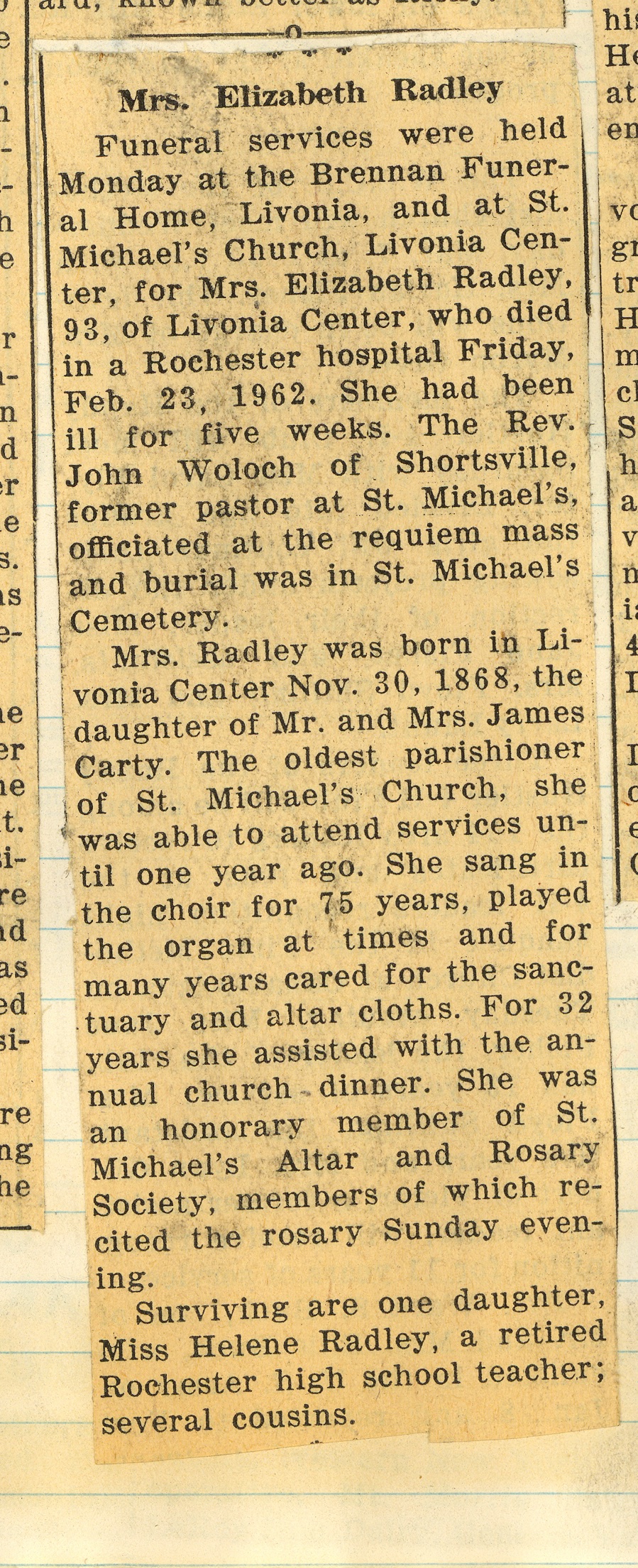This portrait-shaped image appears to be a screenshot or photograph of an old newspaper clipping, primarily in black text against a yellowed background, suggesting age. The clipping features the obituary of Mrs. Elizabeth Radley. Funeral services were held on Monday at the Brennan Funeral Home in Livonia and at St. Michael's Church in Livonia Center for Mrs. Elizabeth Radley, 93, who passed away in a Rochester hospital on Friday, February 23, 1962, after an illness of five weeks. The Reverend John Welch of Shortsville, a former pastor at St. Michael's, officiated the Requiem Mass, and the burial took place in St. Michael's Cemetery. Born on November 30, 1868, in Livonia Center, Mrs. Radley was the daughter of Mr. and Mrs. James Carty. She was the oldest parishioner of St. Michael's Church and actively participated in church services until a year before her death. Notably, she sang in the choir for 75 years, occasionally played the organ, and cared for the sanctuary and altar cloths over many years. Additionally, she assisted with the annual church dinner for 32 years and was an honorary member of St. Michael's Altar and Rosary Society, whose members recited the rosary on Sunday evening. She is survived by her daughter, Miss Helene Radley, a retired high school teacher from Rochester, along with several cousins.